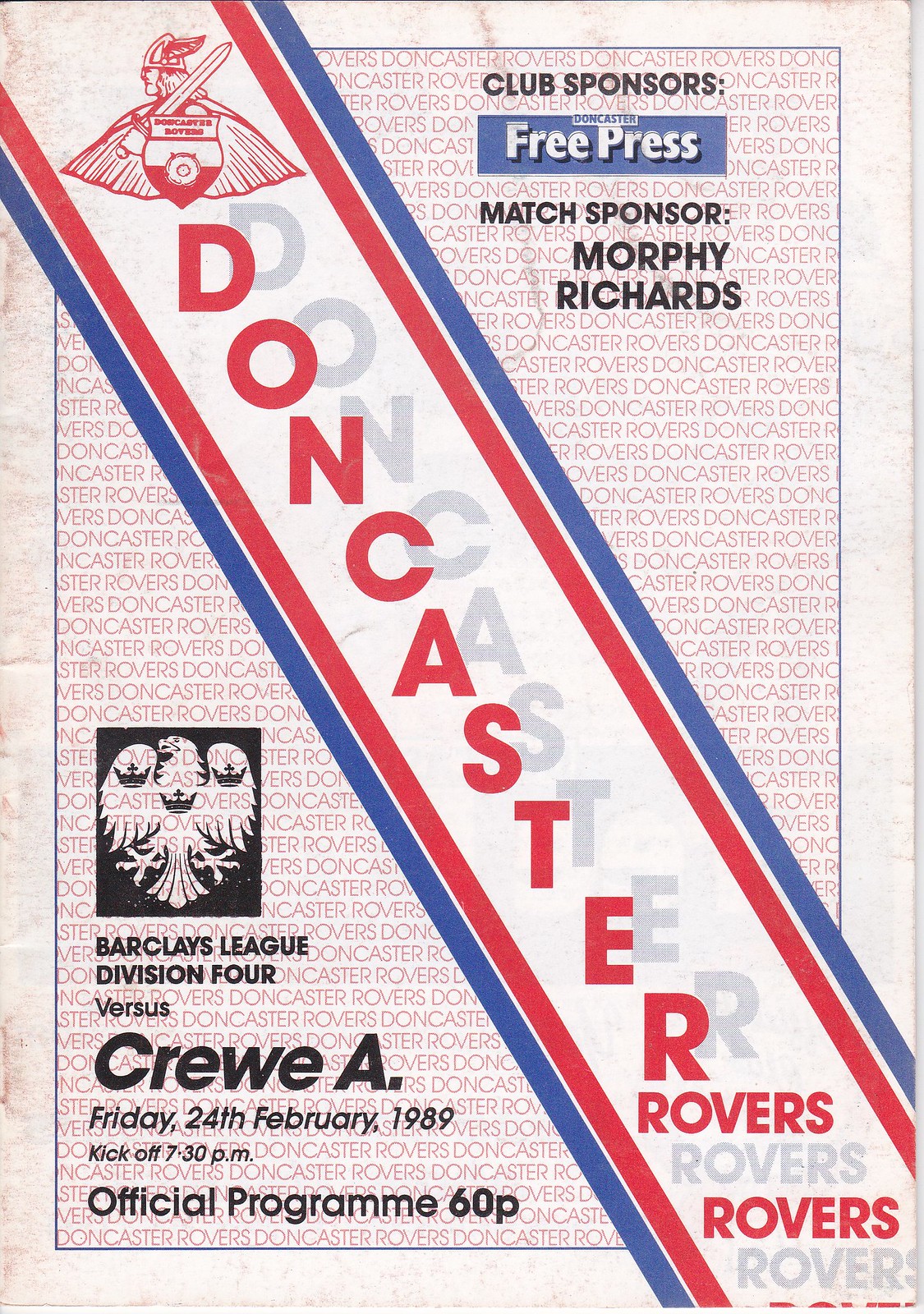The cover of the water-stained and scuffed sports program for the Doncaster Rovers is enclosed in an off-white background that has aged to a light yellowish tone. Dominating the design is a white, diagonal banner with red and blue stripes running from the top left corner to the bottom right corner. This banner bears the prominently displayed name "Doncaster" in large red letters, each shadowed in light gray, and "Rovers" alternately in red and gray. At the very top center of the banner, the team’s red logo, resembling a Viking with a sword, is visible.

The top half of the cover features additional text within various rectangles: a blue box states "Club Sponsors," while another blue rectangle with white text reads "Free Press." Nearby, bold black text announces "Match Sponsor, Morphe Richards." On the bottom left, a crest with a black background and white phoenix bearing two crowns signifies the team’s emblem. Below the crest, key details about the game are provided in black text: "Barclays League, Division 4, versus Crew A, Friday, 24th February, 1989," with a small note at the bottom "Kick off 7:30 p.m." The program price is marked at "60p" in the corner, labelled as the "Official Program."